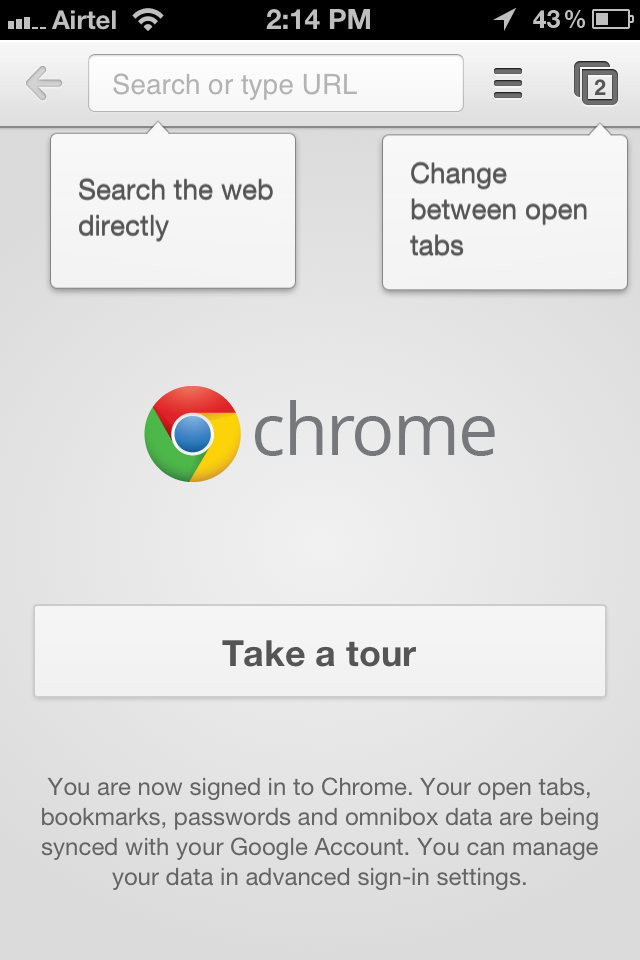The image depicts a smartphone screen displaying the Google Chrome browser interface. At the top section of the screen, which has a black background with white text, the status bar shows various indicators. On the left side, there is the Wi-Fi signal icon and the network name "Airtel," followed by the Wi-Fi strength symbol. Centered in the status bar is the time, "2:14 PM," and on the right side, an arrow pointing right and the battery life indicator showing 43% remaining. 

Below the status bar, the interface transitions to a gray background. On this section, a left-pointing gray arrow is present next to a gray-outlined white search box containing the text "Search or type URL" in gray font. Accompanying the search box is an icon with three gray lines and a double-box symbol with a number "2" inscribed in white within the upper right corner.

The main body of the screen contains two sections: one prompt that says "Search the web directly" within a white square, and another that says "Change between open tabs," also within a white square. These prompts are part of the setup or instructional overlay.

Further down, there is the recognizable Google Chrome logo featuring intertwined segments of orange, green, yellow, and blue forming a circle. Adjacent to this logo, the browser name "Chrome" is written in gray font. Below this text, there is a gray rectangle with the option "Take a tour" written in black font at the center. At the bottom of this section, gray text reads, "You are now signed into Chrome. Your open tabs, bookmarks, passwords, and Omnibox data are being synced with your Google account. You can manage your data in advanced sign-in settings."

The screen provides a comprehensive snapshot of the Google Chrome browser interface on a mobile device, highlighting various functionality tips and user status information.